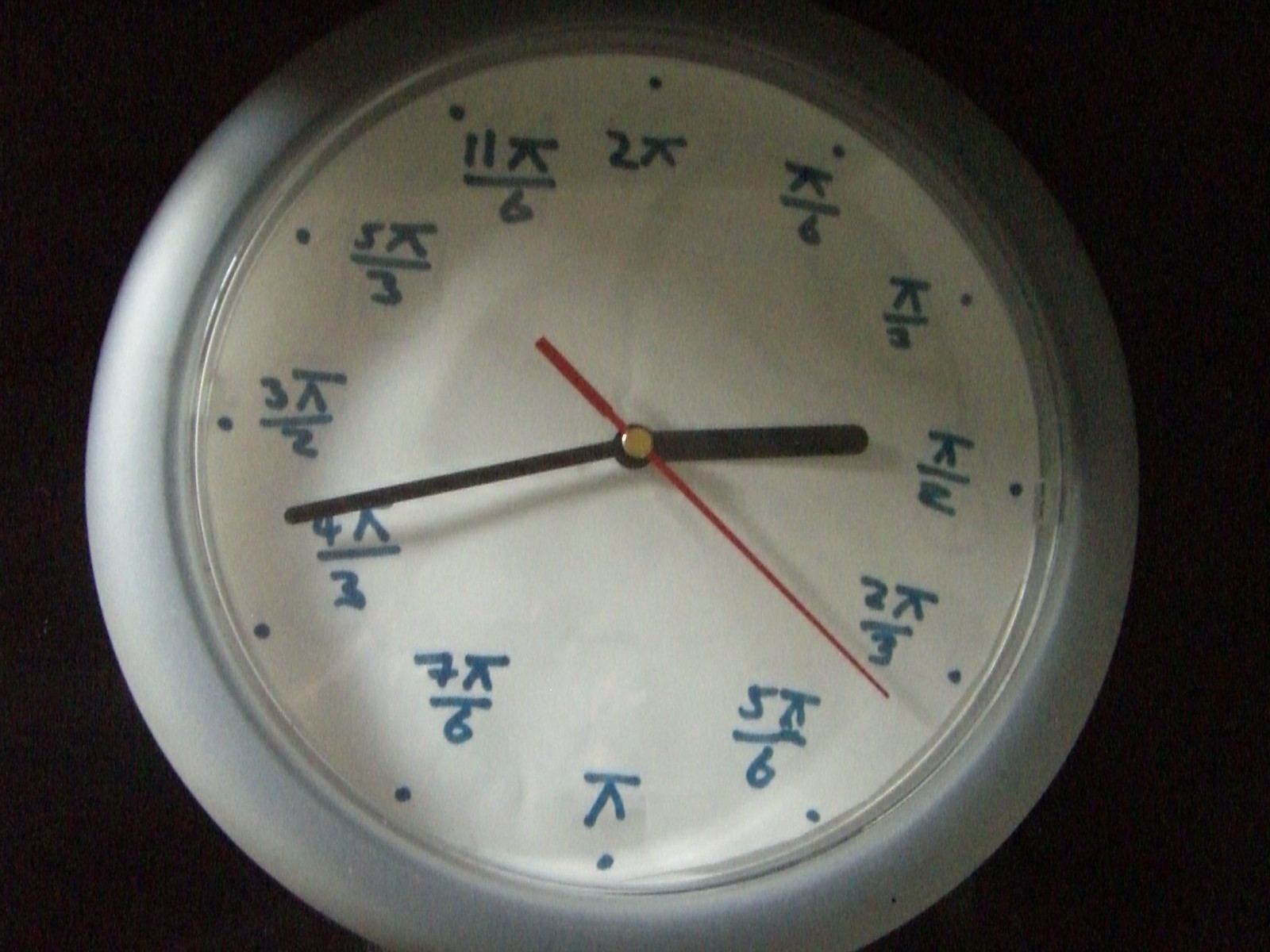The rectangular image prominently features a round clock occupying the majority of the frame, leaving only narrow sections on the left and right sides, with a black background providing sharp contrast. The clock boasts a sleek, silver-gray frame encircling a white clock face. The appearance of the face suggests a crafted, homemade design akin to having been made from a piece of paper. Notably, the numerical indicators on the clock face are expressed through mathematical formulations, which frequently include a symbol resembling a line with an inverted V beneath it. The clock’s hands are stark black, while the second hand adds a pop of color in vivid red.